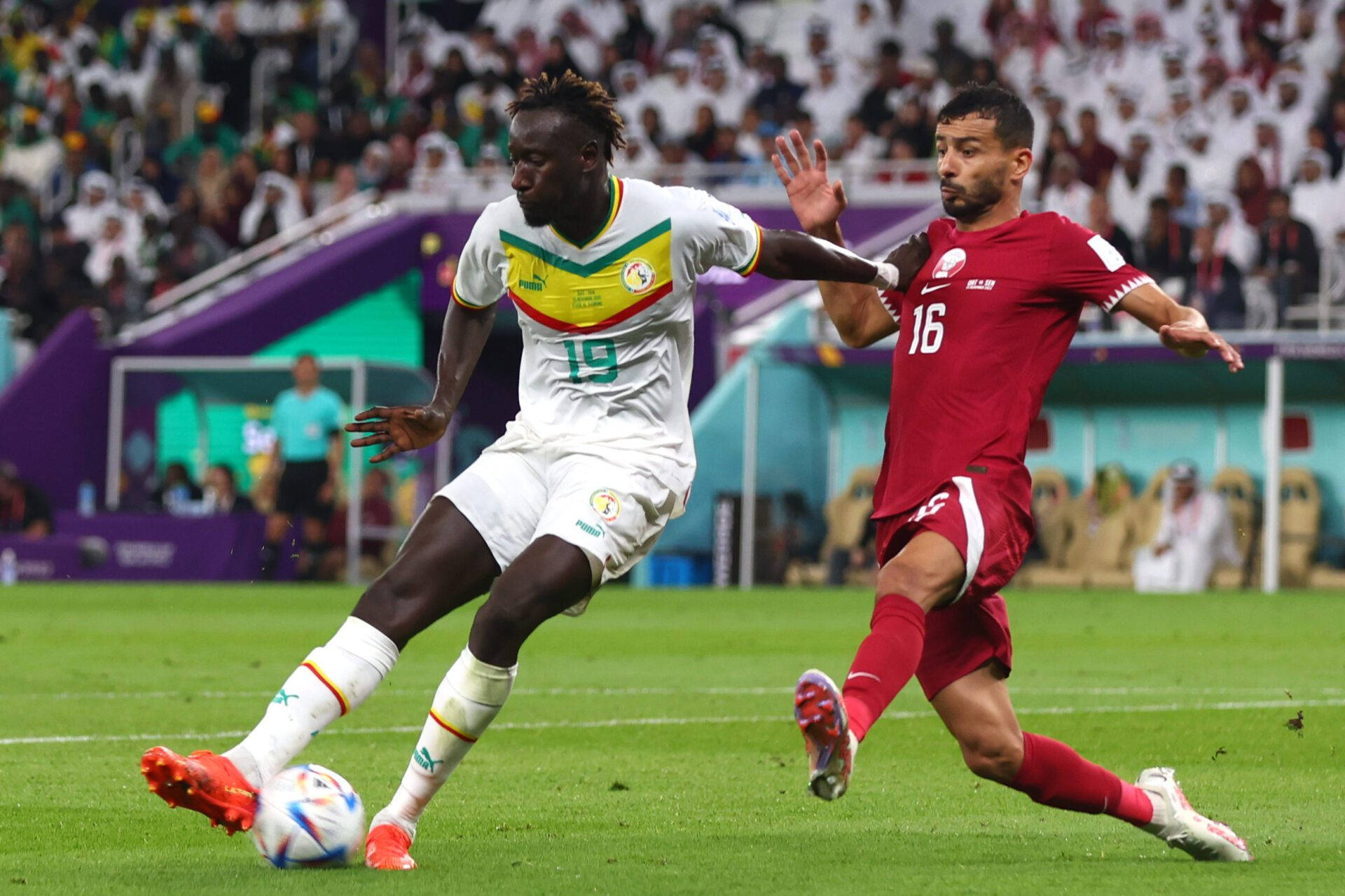This action-packed photograph captures two soccer players from opposing teams amidst an intense match on a grassy field. The player on the left, a black man, is wearing a predominantly white uniform, marked with the number 19 in green-teal on his belly. His shirt features a striking design with a large yellow stripe across the chest, bordered by a smaller green stripe on top and a red stripe underneath. He is equipped with bright orange cleats and white socks trimmed with yellow and red stripes. Positioned with the soccer ball between his legs, he leans backward, both feet turned outward, preparing to kick. His left hand is extended backwards, while his right hand reaches forward, emphasizing the dynamic motion.

Behind him, to the right, is an Indian-looking player characterized by his beard and black hair. Dressed in a vivid red uniform with the number 16 in white on his chest, this player also sports matching red shorts with a white stripe, red socks bearing a Nike emblem, and white cleats. His left leg lunges forward in an attempt to dispossess the ball, while his right leg trails behind in a powerful stride.

Both players are in full sprint on a vibrant green soccer field, their focus and athleticism captured brilliantly. In the background, a blurred stadium filled with spectators and a dugout adds to the lively atmosphere, highlighting the excitement and competitive spirit of the match.